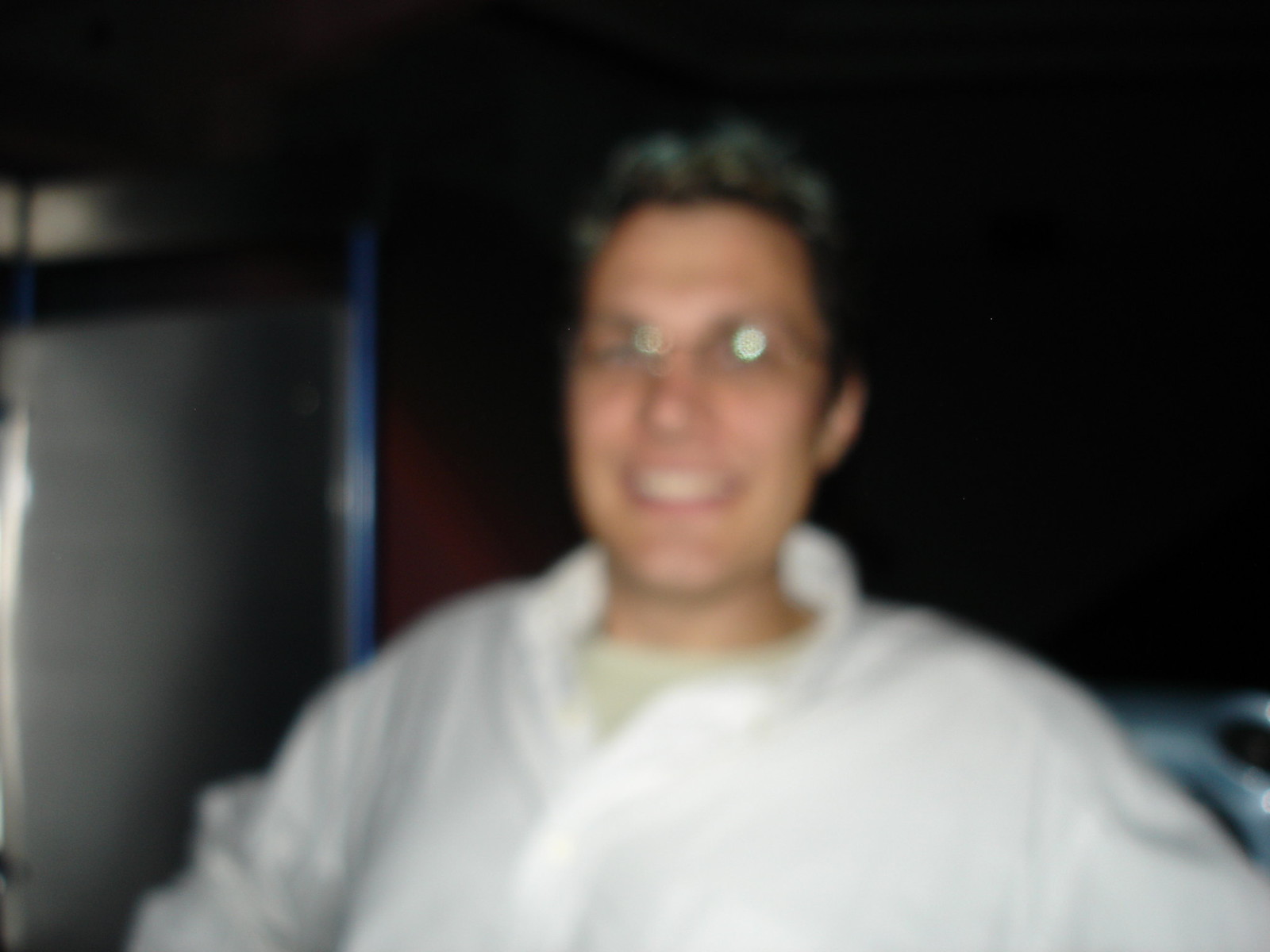The image is an extremely blurry photograph of a middle-aged man, likely in his late 30s or early 40s, characterized by some visible gray in his short, full hair. He is grinning widely at the camera, revealing his teeth in an open-mouthed smile. His glasses are reflecting the camera's flash, resulting in noticeable white spots over his eyes. He is dressed in a white dress shirt with a collar, under which a slightly yellowish or cream-colored t-shirt is partially visible. The background is dark, predominantly black, with a hint of red and a silver rectangular shape on the left side, although the exact nature of these elements is unclear due to the image's poor focus.